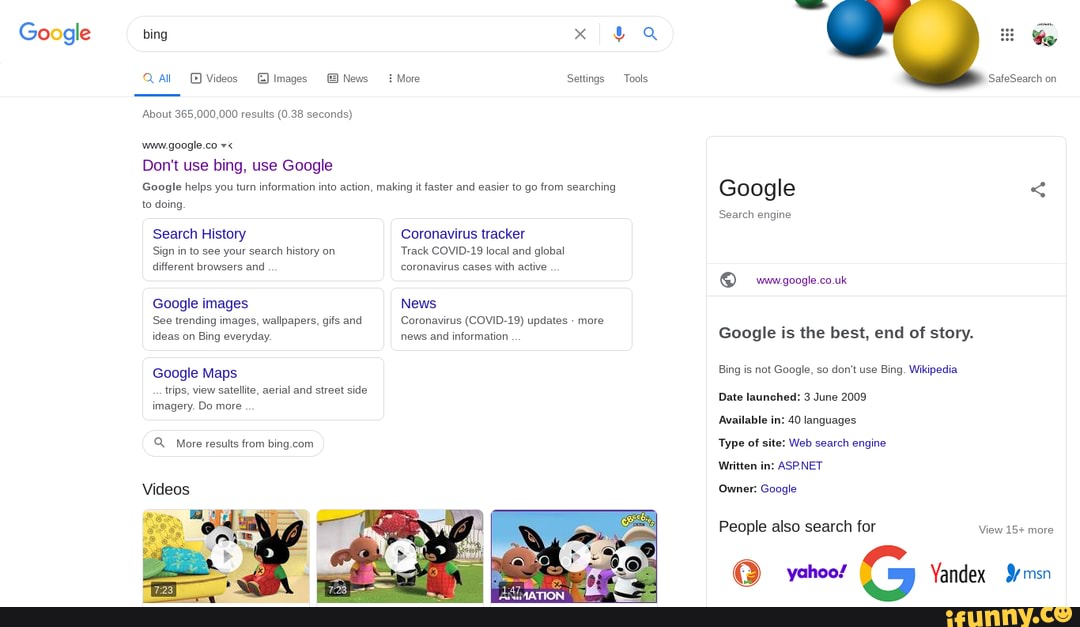The image caption depicts a colorful and detailed graphical interface, featuring various elements related to search engines and their functionalities. At the top, the central focus is on the word "Google" displayed in vibrant colors. Below this, there is a rectangular section with rounded sides resembling circles, which contains the word "Bing" on the left and an "X" on the right. Inside this section is a blue magnifying glass icon followed by three distinct colored balls—blue, red, and yellow—with accompanying symbols and tiny, unreadable text.

Underneath, a magnifying glass icon appears next to an unclear letter in blue, followed by a horizontal line. Adjacent to this is a square with internal content that's difficult to discern. Nearby, there are more small, illegible words and symbols resembling a window and a clock.

Further down, the text "www.google.com" is partially visible with additional unreadable text. A prominent message in purple reads, "Don't use Bing, use Google." There are several grey-outlined boxes labeled "search history," "coronavirus tracker," "Google Images," "news," and "Google Maps." Below these, there's a section with cartoon images of a bunny and its friends labeled "videos."

On the right side, another grey-outlined box reads "Google search engine," accompanied by a share symbol and a planet icon. Purple text, too small to make out, states "Google is the best, end of story," followed by more unreadable words.

At the bottom, the phrase "people also search for" precedes an orange circle with white inside it, featuring the Yahoo logo, the Google "G," and the term "Yandex," with the "Y" in red and the rest in black. The butterfly logo for MSN is also displayed, and a black rectangle at the bottom contains the text "ifunny.c" in yellow beside a smiley face icon.